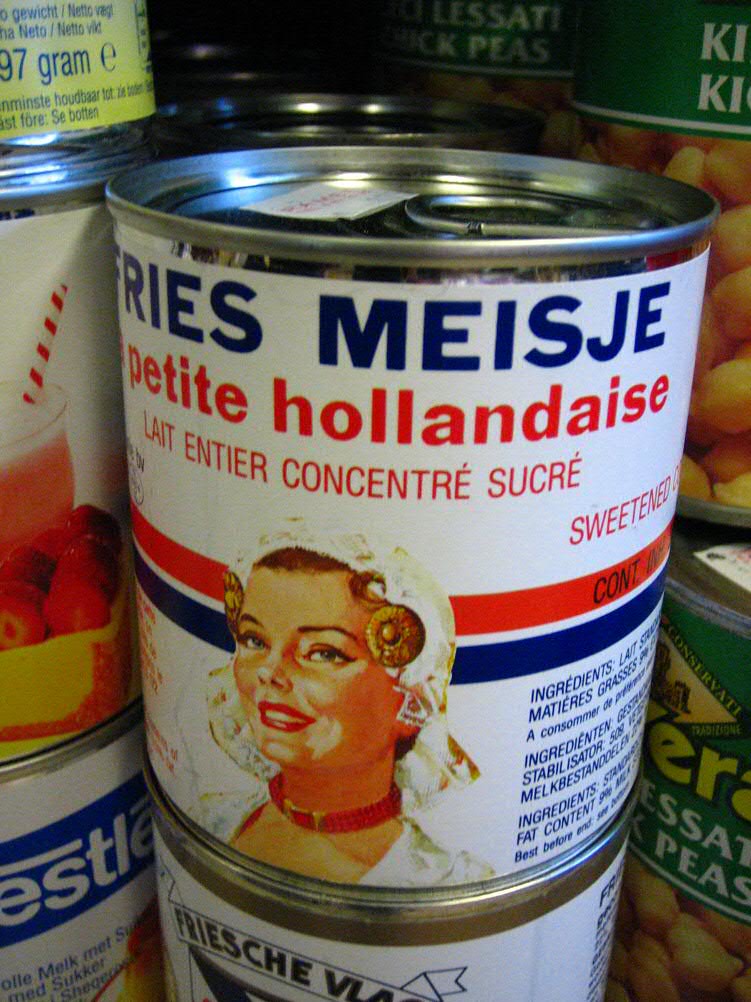The image showcases an old-fashioned kiln, crowned with a silver lid. On the front of the kiln is a white label featuring the illustrated face of a woman adorned with a red collar and a white veil. The label reads "Petite Hollandaise" and includes additional text such as "sweetened." Below this text, there are both a red and a blue rectangle, followed by lists of ingredients in multiple languages including English and Spanish. The scene evokes a rustic, historical charm, with the overall aesthetic suggesting a product from a bygone era. To the right of the kiln, there are images of two cans: one labeled as beans in the upper-right, and another labeled as peas in the bottom-right.